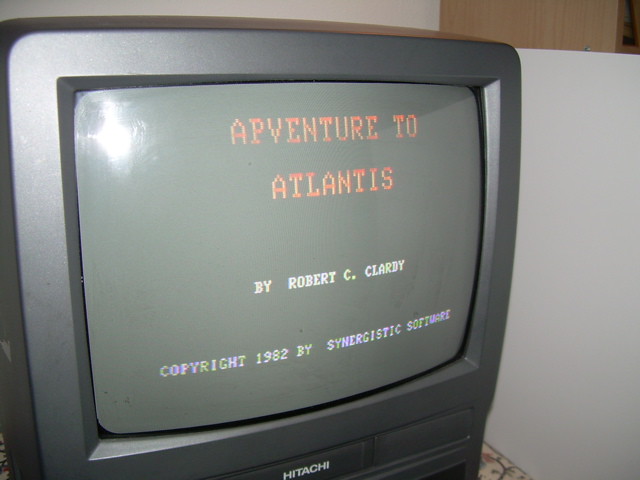This photograph captures a zoomed-in view of a vintage Hitachi CRT television encased in a light gray plastic frame. The TV, positioned against a white wall with a wooden shelf visible at the top, displays a boot-up screen for a video game titled "AP Venture to Atlantis" in pixelated orange text. Just below the title, the text "By Robert C. Clardy" appears in small white capital letters, followed by "Copyright 1982 by Synergistic Software," also in white. The screen seems washed out due to either the old CRT tube or poor lighting conditions, and there's a noticeable light reflection in the upper left corner of the screen. The Hitachi brand name is prominently displayed in small white letters at the bottom of the TV. On the right side of the image, a light gray wall or divider is visible, casting a shadow from the television.